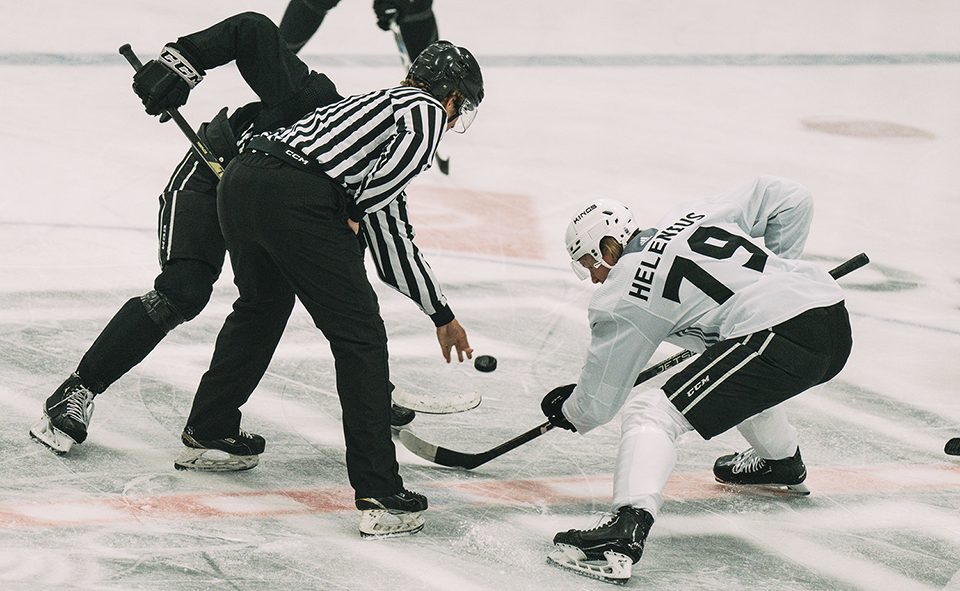The image depicts a lively hockey game captured in a landscape layout, showcasing a dynamic moment where two players are facing off as the referee prepares to drop the puck. The referee, clad in a black and white striped shirt, black pants, and a black helmet, is seen in mid-action with the puck suspended in the air from his left hand. On the right, a player wearing a white helmet, a white jersey with 'Helenius' and the number '79' emblazoned in black, black shorts, white socks, and black skates, is poised for the face-off. Opposing him is a player dressed head-to-toe in black, partially obscured by the referee's position. The ice rink below them is a clean white canvas with red and black accents, all players donning helmets and skates, emphasizing the intensity and uniformity of the scene.